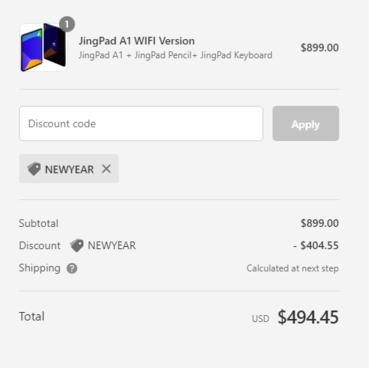**Detailed Caption:**

The image features a promotional advertisement for the JingPad A1 Wi-Fi version. The offer includes the JingPad A1 tablet, along with the JingPad Pencil and JingPad Keyboard, all priced at $899. The advertisement highlights an input field for a discount code, where users can enter "new year" to receive a substantial discount. There is an "Apply" button next to the discount code input field. Once applied, the discount "new year" is shown to reduce the subtotal from $899 to $494.45, providing a savings of $404.55. The shipping cost is calculated in the next step. The total amount after applying the discount is prominently displayed as $494.45. The image showcases the tablet with a sleek design, featuring a white version depicted in a gray circle above a background photo showing the tablet's screen. The advertisement also includes a vibrant color palette with blue, green, orange, gray, black, and white accents, enhancing its visual appeal. This promotion offers a great deal on a high-quality tablet bundle.